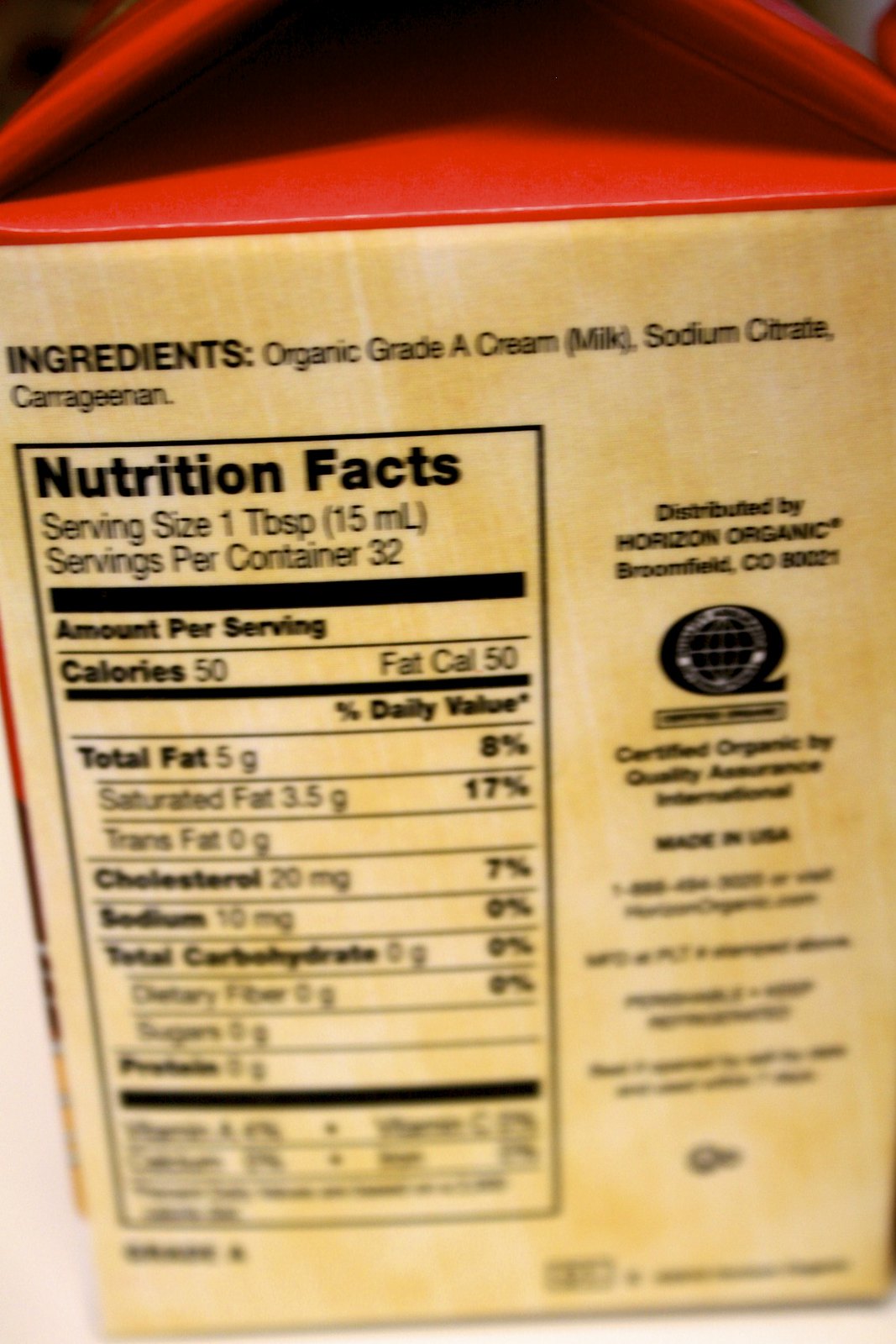This is a color close-up photograph of a carton of dairy cream. The focal point of the image is the panel displaying the nutrition facts and ingredients. The carton is a light, dusty pink with subtle yellow undertones, giving it a vintage yet refreshing appearance. 

At the top of the panel, the ingredients are clearly listed as organic grade A cream, milk, sodium citrate, and carrageenan. The nutrition facts indicate that a one-tablespoon serving contains 50 calories, 5 grams of fat, and 3.5 grams of saturated fat. Unfortunately, the remainder of the nutritional information is blurry and out of focus, making it difficult to read.